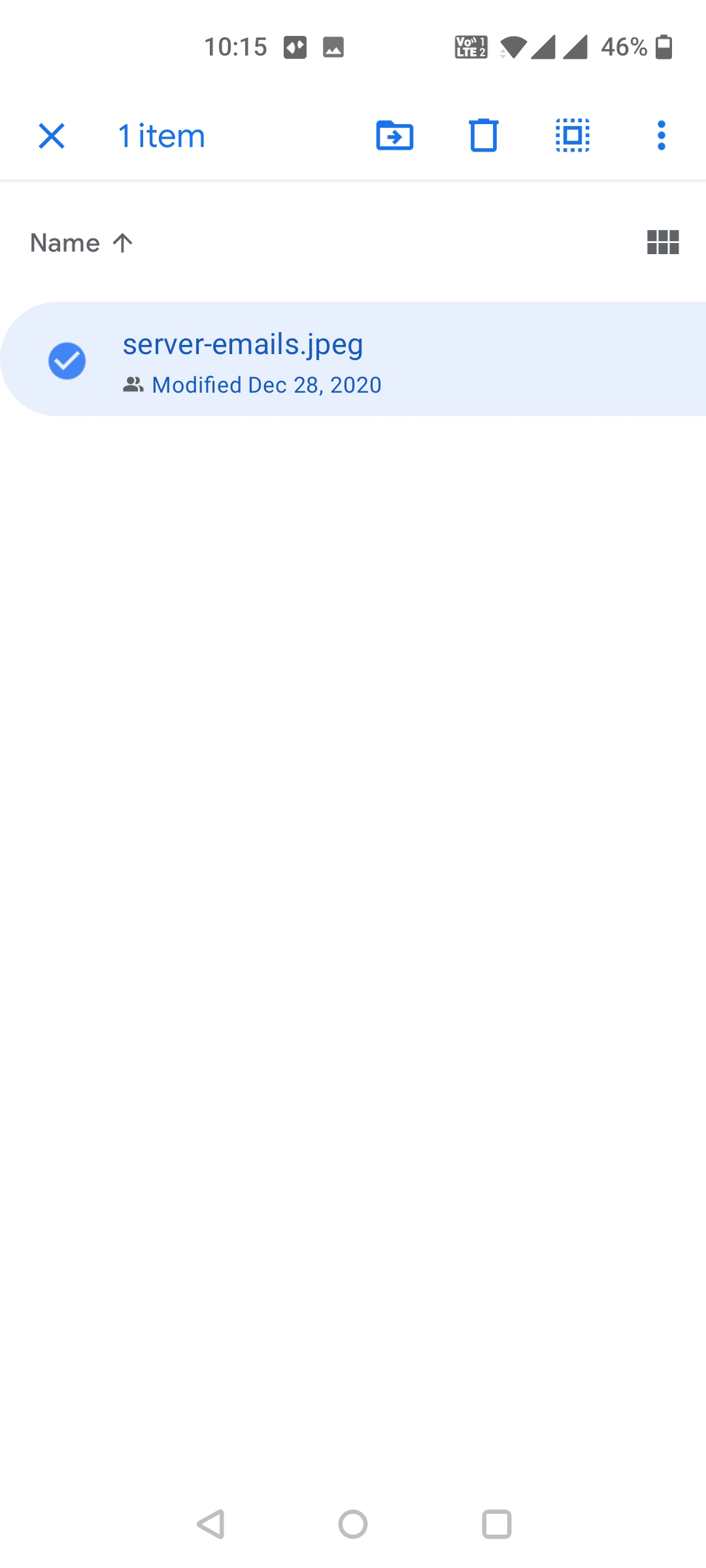The image depicts a smartphone screen showing a file management interface. It is currently 10:15 AM, as indicated on the left side, with the battery level at 46% on the right side along with icons for cell signal strength, Wi-Fi, volume, and brightness controls. Below this status bar, a blue header contains an 'X' on the left, indicating an option to close or exit, and says "1 item" next to file action icons for moving to a file and deleting (garbage icon). 

The central part of the screen displays a section with a dashed-outline box and a menu icon represented by three vertically stacked dots. Underneath, there is a sortable column header labeled "Name" with an upward arrow indicating ascending order. The file listed is "server email.jpg," which was modified on December 28th, 2020. This entire section is contained within a curved rectangle ending abruptly on the right side of the screen. The background is a light blue color with dark blue font, and a circle with a check mark appears next to the file name, indicating selection.

Above the file information, there are two rows of three small black icons each, adding to the interface's functionality. The bottom portion of the screen consists mainly of white space, roughly three times the area of the file display section. The navigation bar at the very bottom includes icons: a back arrow, a home circle, and a recent apps square.

The overall color scheme in the interface includes gray, white, blue, and black tones.